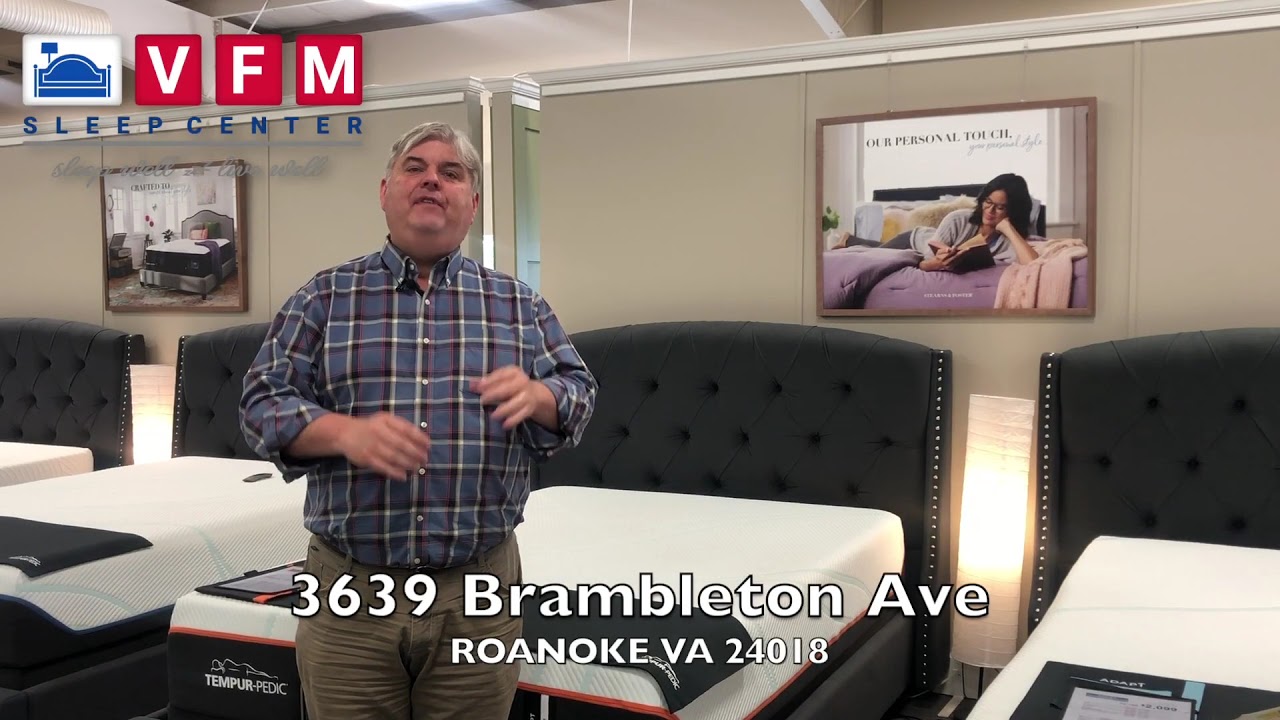This image captures a moment inside a spacious showroom, likely taken from a TV commercial for a bed retailer. A slightly overweight man with silver hair, dressed in a long-sleeve blue checkered shirt with white buttons and dark brown pants, stands prominently in the center. His upper body, face, and legs up to his knees are visible. The man appears to be in mid-speech, his hands slightly blurred due to movement.

Behind him, a row of four beds with white mattresses stretches along a cream-colored wall. The bed closest to the man is fully visible, while the others are partially obscured. These beds feature green headboards adorned with embroidery and buttons, giving them a majestic yet uniform appearance.

The room is adorned with framed paintings of beds, enhancing the theme. In the upper left corner of the image, a small blue bed icon sits within a white box next to red squares containing the letters "VFM," followed by "Sleep Center" in blue text. Additionally, the address "3639 Brambleton Avenue, Roanoke, VA 24018" is clearly displayed in white text at the bottom center of the image.